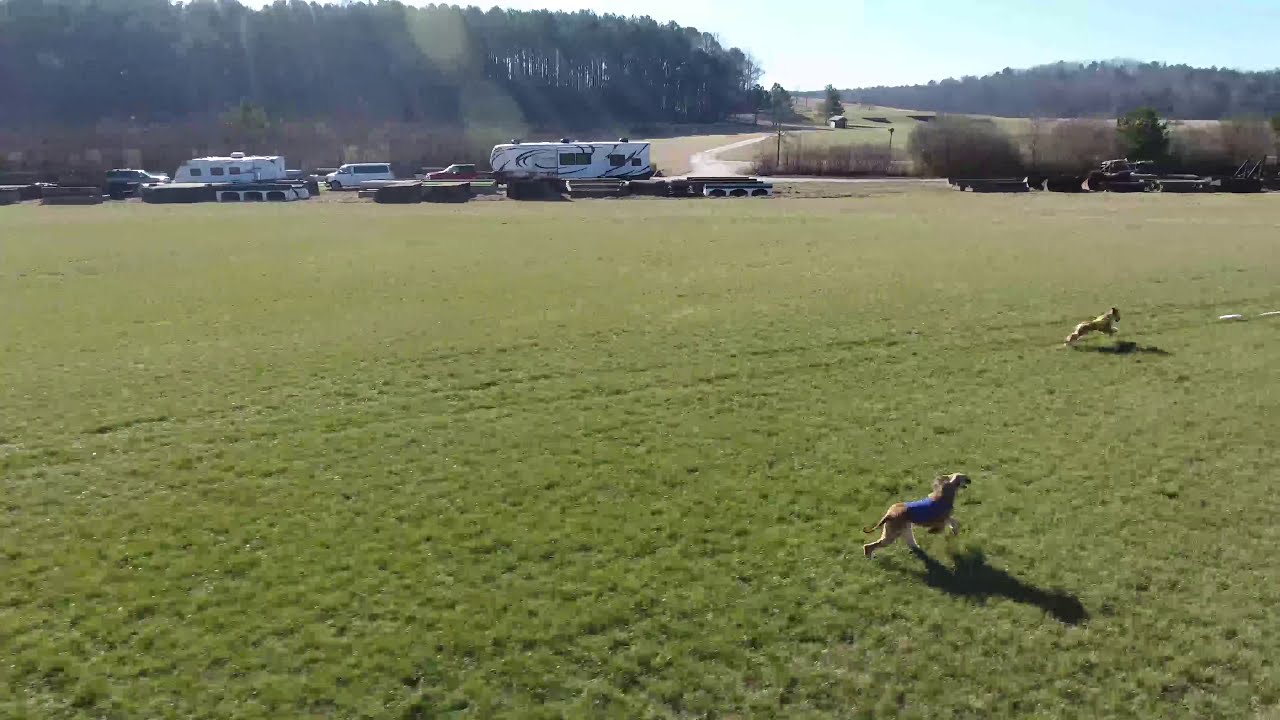The image is a color landscape photograph, likely taken from a drone on a bright sunny day. The foreground features two small breed dogs joyfully running across a well-maintained grassy field. One dog, closer to the photographer, wears a blue vest, while the other is slightly further back and running to the right. Shadows of the dogs elongate towards the photographer, enhancing the sense of movement. In the background, there are about two or three large white RVs along with several other vehicles parked near a dirt road. This road extends horizontally and then meanders into the distance, leading to more fields and low-lying hills adorned with dense forest and trees. There are no people visible in the image, emphasizing the serene and open nature of the scene.